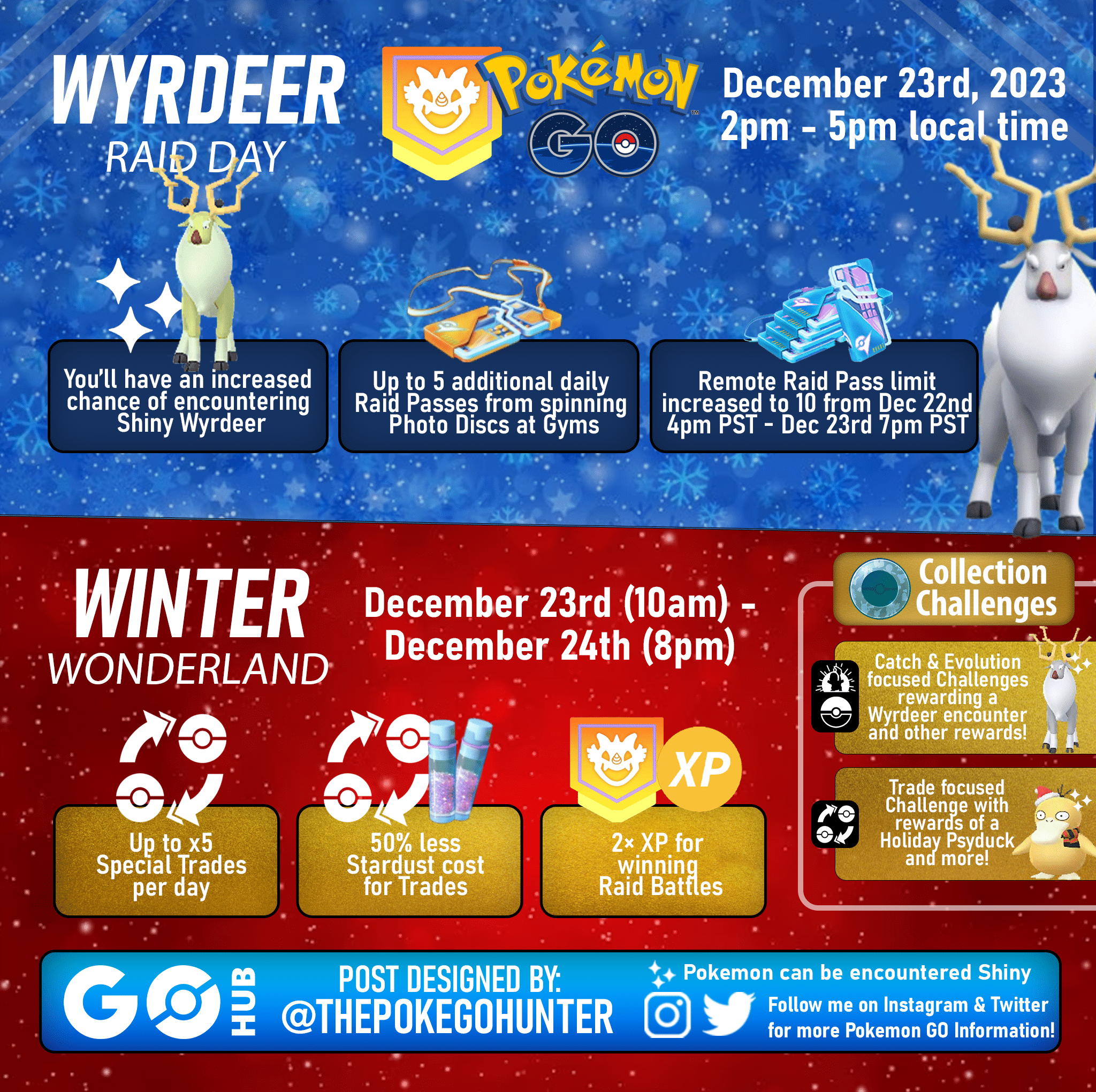**Caption:**

This advertising banner is for a Pokémon GO event with a festive Christmas theme. The background is divided diagonally, with the top half in red and the bottom half in a snowy overlay featuring snowflakes. The title, "Weird Deer Raid Day," is prominently displayed, indicating a special raid event taking place on December 23rd, 2023, from 2 p.m. to 5 p.m. local time. Surrounding the title are images of deer-like Pokémon, flanking the header with festive adornments.

The banner is divided into sections to highlight various features of the event:

1. **Event Details:**
   - **Increased Shiny Encounter Rates:** Players will have a heightened chance of encountering a shiny version of the Pokémon "Weird Deer."
   - **Raid Passes:** Participants can gain up to five additional daily raid passes by spinning Photodiscs at gyms.
   - **Remote Raid Passes:** The limit for remote raid passes increases from 10, starting from December 22nd at 4 p.m. PST to December 23rd at 7 p.m. PST.

2. **Winter Wonderland:**
   - This sub-event runs from December 23rd at 10 a.m. to December 24th at 8 p.m., featuring unique gameplay bonuses, distinguished by yellow boxes with informative icons.

3. **Social Media Engagement:**
   - At the bottom, the banner credits the design to "Go Hub" and the user @ThePokeGoHunter. It also notes that certain Pokémon can be encountered as shiny versions during the event.

The banner encourages players to follow on Instagram and Twitter for more Pokémon GO updates, with respective icons featured prominently.

---

This detailed breakdown captures the key aspects of the advertisement, making it easy for viewers to understand the event's highlights and how to participate.